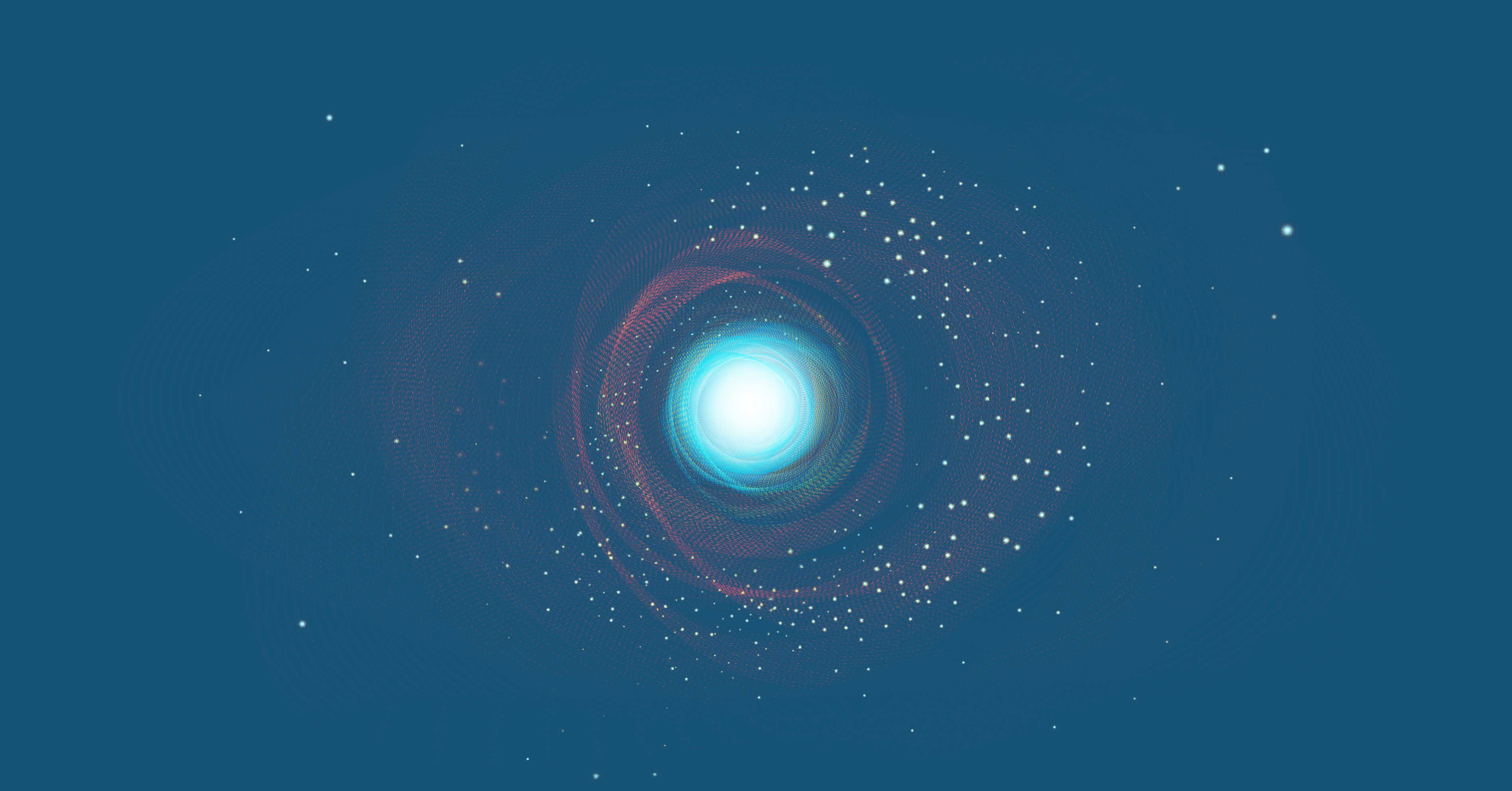The image is a detailed digital artwork depicting a dazzling galaxy set against a flat, dark blue background symbolizing the vast expanse of space. At the center of the composition is a bright, radiant orb from which luminous light beams emerge. This central light source is encircled by swirling clouds and several faintly colored whooshes, predominantly red and pink, gradually blending into yellow as they spiral inward, pulled by the immense gravitational force of the galaxy. Dotted throughout the scene are varying sizes of white spots, representing distant stars, that become denser as they approach the central bright sphere. The overall shape of the galaxy is distinctly circular with these intricate spirals, and the stars tend to cluster more near the center, enhancing the intensity of the central luminous area. The image is rectangular, with the width being about twice the size of the height, capturing the majestic and mesmerizing nature of a spiral galaxy in a 2D artistic rendition.